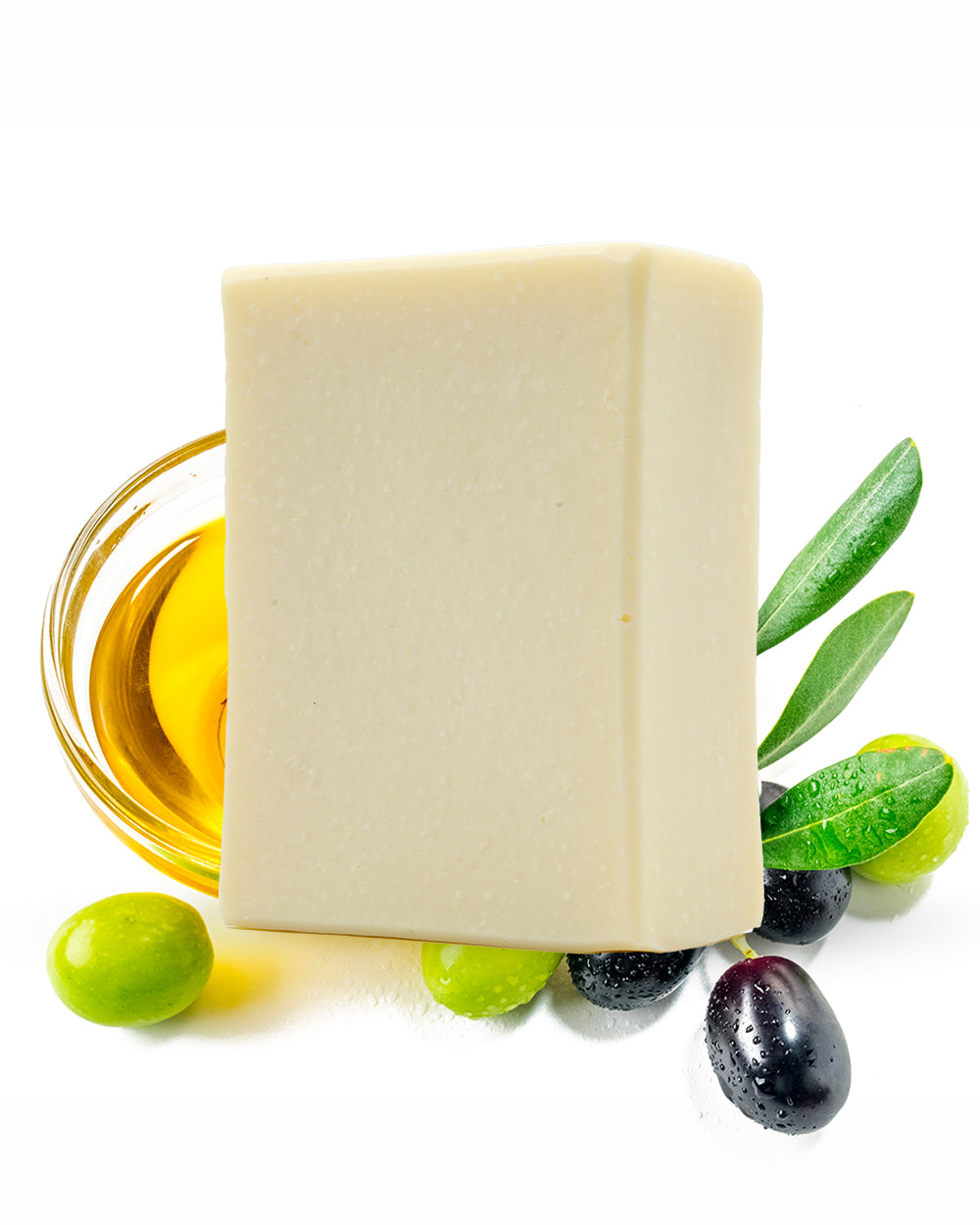The image features a large block of beige-colored cheese, which resembles a bar of soap at first glance. The cheese is positioned centrally against a solid white background, with its vertical rectangular shape prominently displayed. Both the front and one side of the cheese are visible, emphasizing its substantial thickness. Surrounding the cheese, there's an arrangement of wet red and green grapes, all adorned with tiny water droplets, enhancing their fresh appearance. Specifically, a couple of somewhat purple-hued red grapes lie below the cheese, while three green grapes are scattered around—one to the far right, one in the middle, and one to the left. Three green leaves also peek out from behind the cheese, similarly covered in water droplets. Partially beneath the cheese, there is a small glass condiment dish containing a yellow liquid, which could be vegetable oil, honey, or lemon juice. The lighting in the image causes the top of the cheese to appear brighter, gradually becoming a bit darker towards the bottom, with shadows evident around the elements on the right and bottom of the composition.